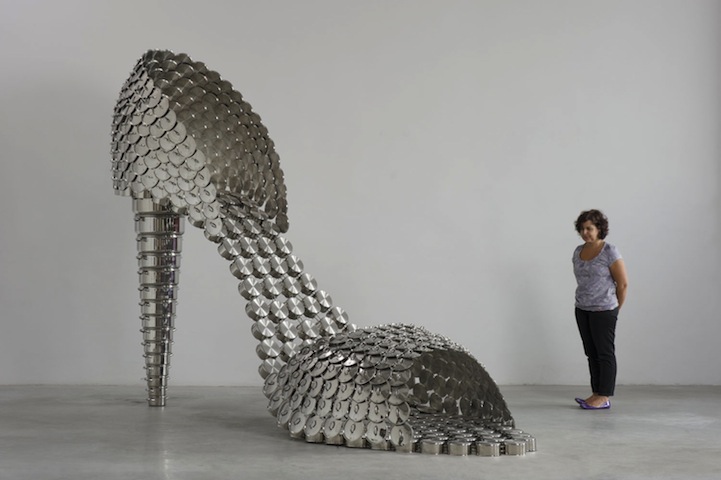In an indoor gallery setting with polished concrete floors reflecting the artwork, stands a giant, intricate piece of contemporary art in the form of a high-heeled shoe, made from circular metal parts resembling pens and pots. The shoe, with an open toe and a very high, thin heel almost like a stiletto, is strikingly silver and smooth, spanning about two to three inches in length and towering over a woman who stands beside it. The artwork, which emphasizes its stature and detailed craftsmanship, reaches twice the height of the woman. She stands to the right of the shoe, slightly facing it, with short, brown, curled hair that falls to her shoulders. She appears to be in her 60s, dressed in a light purple scooped-neck, short-sleeved shirt, black pants, and purple flats. Her hands are placed behind her back as she gazes at the impressive metallic structure. The background features a light gray wall, which together with the reflective floor, complements the contemporary aesthetic of the sculpture.